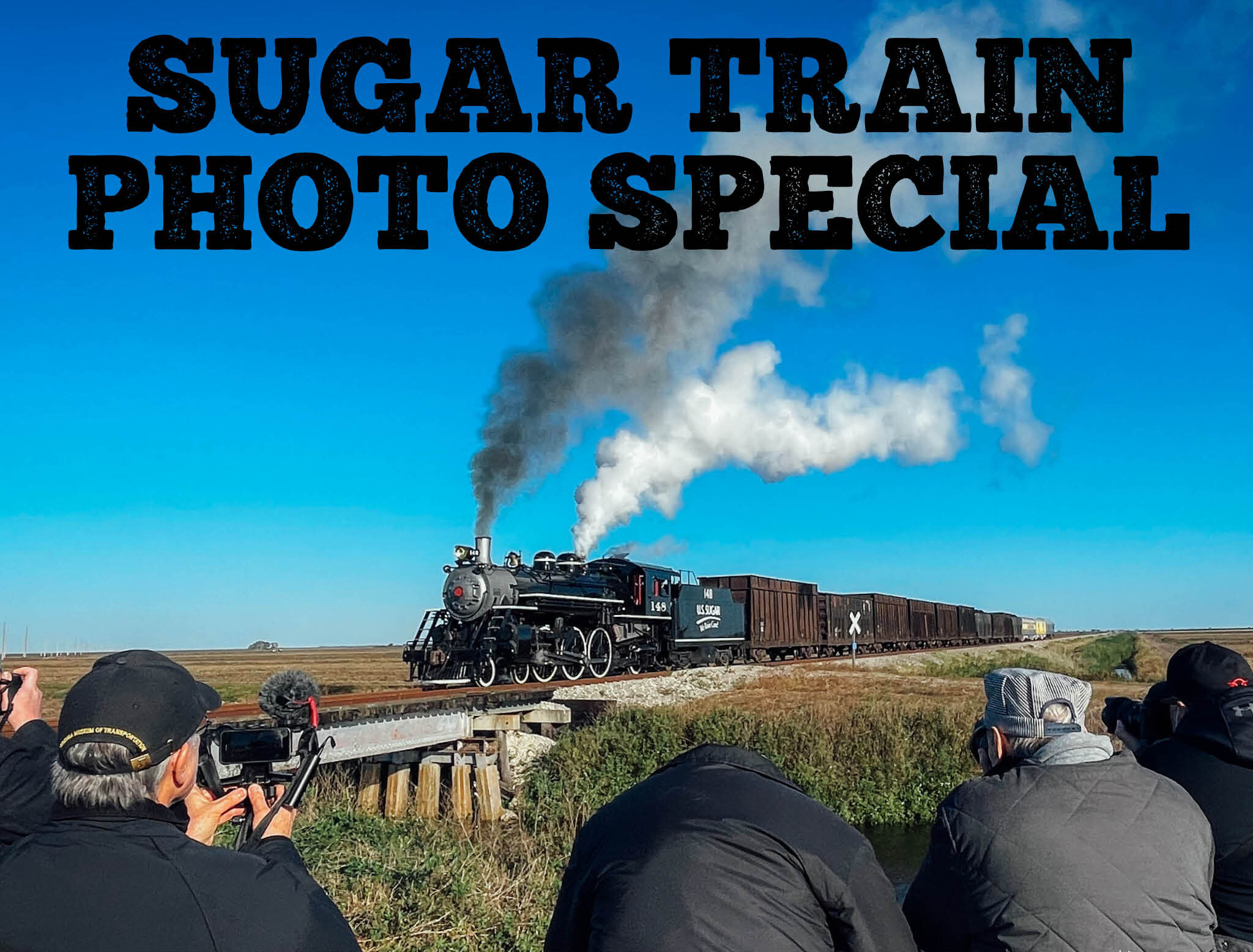The image is a color photograph in landscape orientation, capturing a charming scene of an old-fashioned steam train crossing a small bridge in the middle of a vast, flat, grassy field. The steam engine and its wooden cargo cars dominate the center of the image, chugging towards the left, with two distinct plumes of smoke—one gray at the front and another white slightly behind it—rising into the clear blue sky. This train, clearly marked for a special event, has "Sugar Train Photo Special" written in bold black text at the top of the picture. In the foreground, a group of three or four people, positioned at the bottom of the image, are eagerly taking photographs of this nostalgic scene, their cameras pointed towards the approaching train. A tiny valley and the bridge beneath the tracks add further depth to this scenic and representationally realistic photograph.